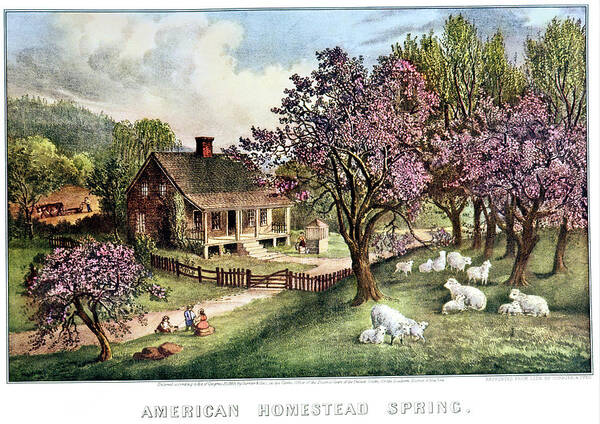This is a high-quality, colorful charcoal drawing set in the 1800s, evoking a cheery and textured Victorian style. It depicts an American homestead in the springtime, characterized by a large brown wooden house with a V-shaped roof and a little red chimney. The house features a spacious deck with an awning, supported by wooden steps that lead to the porch. A prominent, large wooden fence with a gate encloses the entire homestead, which is surrounded by various types of trees, including vibrant cherry blossom trees with pink leaves.

In front of the house, a well sits on the grassy path leading up to the entrance, where a group of people is visible. This group includes a lady in a red dress, a cowboy in blue jeans and a white shirt, and a small child beside them. They appear to be seated near the dirt path that borders the house. To the right, a flock of sheep, with both adults and lambs, are grazing and resting under the cherry blossoms.

On the left side of the image, a mule pulls a plow navigated by a farmer, working diligently in a field that transitions into a wheat field of golden hues. The backdrop features rolling hills or mountains under a cloudy, yet cheerful, blue sky. This idyllic, detailed scene encapsulates rural life in the 1800s with its vibrant and textured depiction.